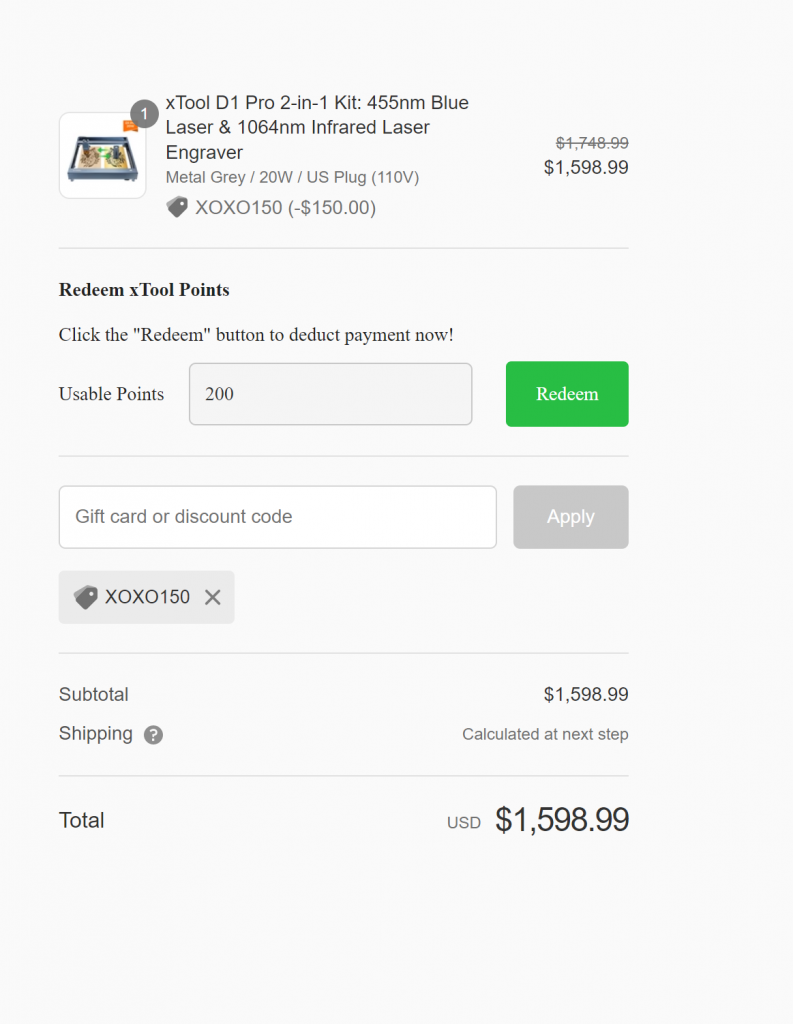The screenshot captures a checkout page for an item, specifically the "X-Tool D1 Pro 2-in-1 Kit". The item is prominently displayed at the top left corner of the page, accompanied by a small image of the laser engraver. This image is marked with a gray circular badge at the top right, displaying the number "1" to indicate the quantity. 

On the left of the item name, the price is listed. Initially, the cost was $1,748.99, but it has been discounted to a new price of $1,598.99, with the original price crossed out. 

Below the item's image, title, and price, there's a feature for the user to redeem any available tool points. The interface shows the user has 200 usable points, displayed in a box. To the right of this box, a green button with the text "Redeem" in white allows users to apply their points.